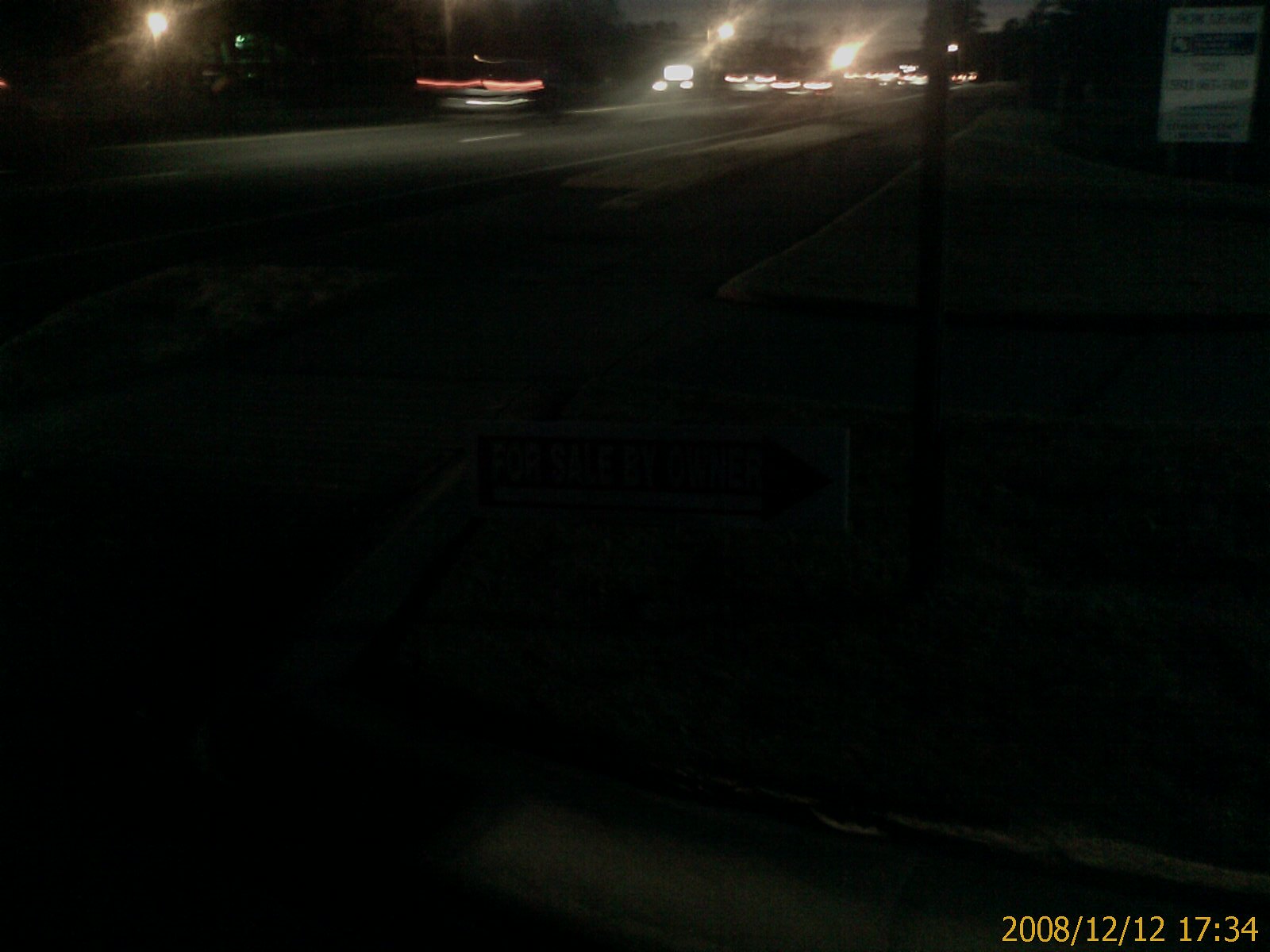The image depicts a somber and dimly illuminated intersection where two highways converge. At the bottom of the image, a row of numbers, likely a date, is visible. In the distance, the headlights of numerous vehicles create a trail of lights, suggesting heavy traffic coming towards the viewer. The multi-laned highway extends towards the left. High above, near the top left corner, a very bright light is prominent, perhaps from a streetlamp or traffic light. A string of lights shows up as pink, adding a subtle hue to the scene. In the foreground, on the right-hand side, a narrow post or streetlamp stands, subtly casting light into the dim surroundings.